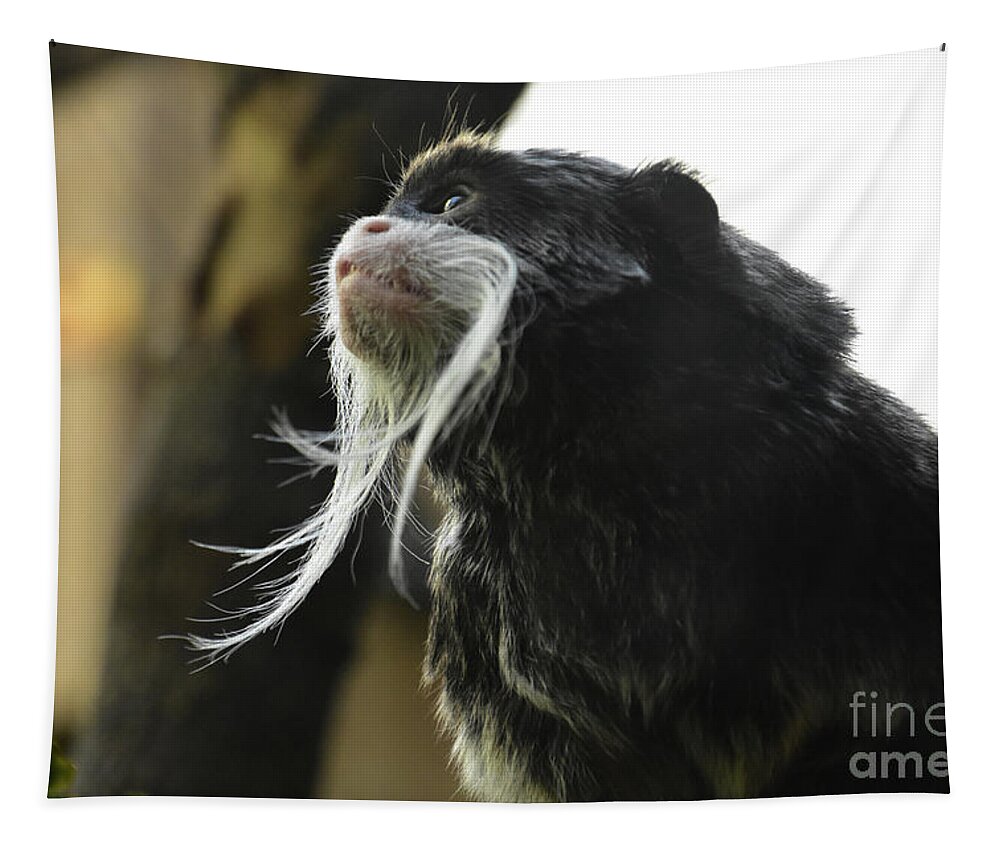This is an image of an Emperor Tamarin Monkey, prominently featured on a duvet cover. The monkey, with dark fur and black head, has a distinctive white snout and extraordinarily large nose holes, giving it a unique appearance. The monkey's muzzle and nose resemble those of a smaller dog, such as a Pekingese or Chihuahua, but what stands out most are the long, white, wispy whiskers hanging Fu Manchu-style from either side of its nose. It is positioned from the bottom right corner to the top left corner of the image, as if squatting with its longer front limbs supporting its stance, almost akin to a cat. The background to the left fades into a tan and brown hue, with some fuzzed out elements that resemble a tree, contributing to its natural setting. The image's surface appears to slope towards the center, suggesting a photograph printed on fabric and hung on a wall. The bottom right corner bears the light lettering “F-I-N-E” followed by “A-M-E,” a watermark indicating Fine Art America, which likely holds the rights to this intriguing depiction of the Emperor Tamarin Monkey.